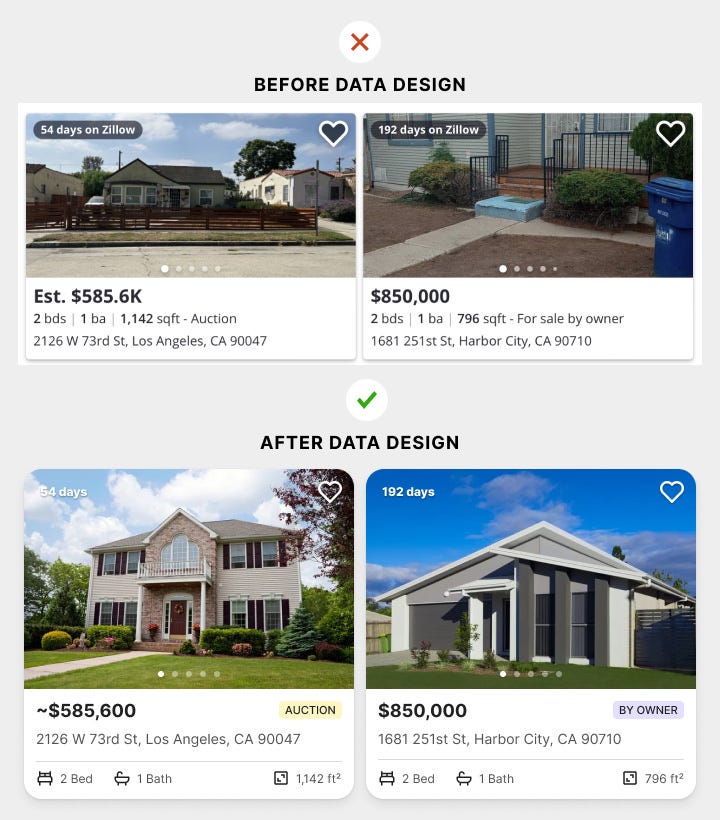This composite image depicts various properties listed on Zillow with several distinct details. 

In the top section, there's a comparative "before” and “after” design of a property marked by red X's. The top-left corner indicates the property has been listed for 54 days on Zillow, followed by a grey heart icon. The property features a fenced yard, lush greenery, and a grassy lawn. It is listed at $585,600. This home has two bedrooms, one bathroom, and spans 1,142 square feet. It's located at 2126 W 78th Street, Los Angeles, CA, 90047, and has been on the market for a total of 119 days.

Adjacent to this, another property is featured, characterized by a fenced yard, steps leading to the entrance, and visible patches of dirt around a blue trash can. This unfinished property is listed at $850,000, with two bedrooms and one bathroom, covering an area of 796 square feet. It is for sale by owner at 1681 251st Street, Harbor City, CA, 90070. 

In the middle, a grey checkmark signifies the "after" design, presenting the property in a more completed state. Beside this, a square indicates it has been listed for 54 days. This building showcases modern architecture with stone walls and a vibrant green lawn, under a bright blue sky. 

Altogether, these detailed snippets offer an array of property listings with insights into design stages, listing durations, and price points, providing prospective buyers with a comprehensive overview.